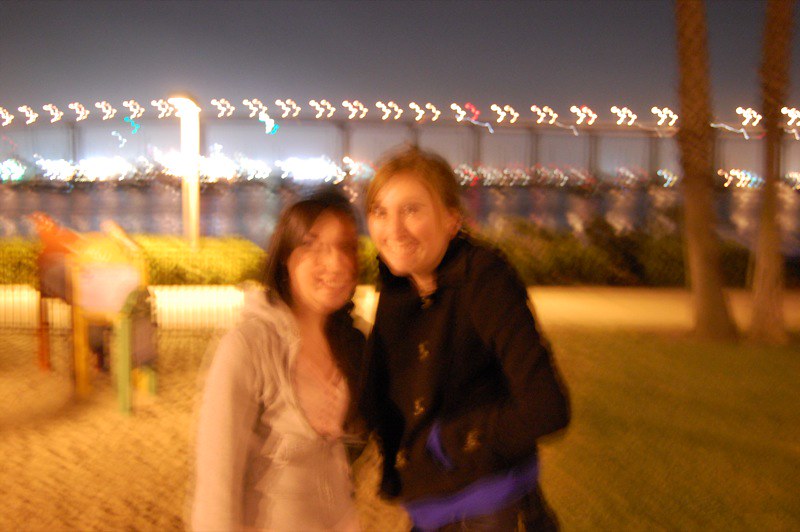In this very blurry photograph, two smiling women stand side by side, both looking directly at the camera. The woman on the right, slightly taller, has sandy blonde hair and wears a long-sleeved black top, possibly with a blue shirt underneath. The shorter woman on the left has darker brown hair and larger glasses, and she is dressed in a beige hoodie. The background features a large, illuminated fence with lighting across the top, suggesting they are in a dimly lit outdoor area. The ground beneath them appears to be either dirt or sand, and there are trees and a stand faintly visible on the left. The overall image quality is fuzzy, making facial details and the exact nature of the surroundings difficult to discern.